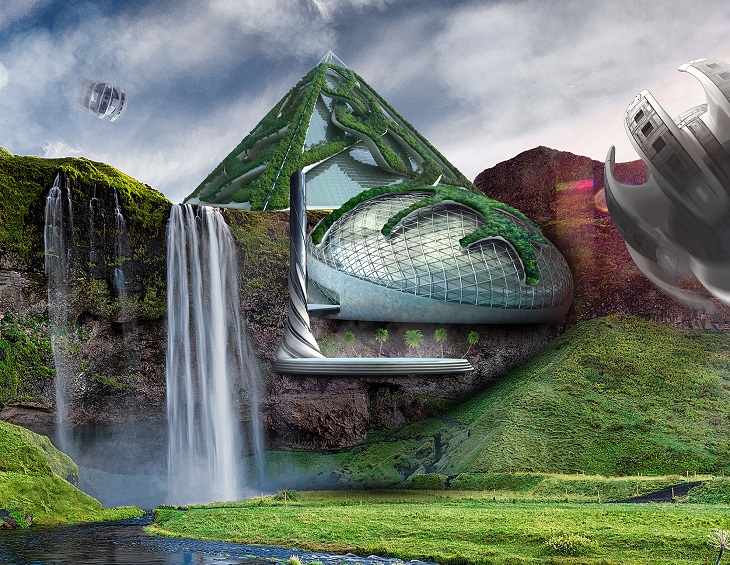This is a highly detailed, computer-generated image depicting a surreal and futuristic landscape. A massive, grassy hill that transitions into rocky terrain and ending in cascading waterfalls dominates the scene. Atop the hill sits a striking glass pyramid adorned with intertwining, braided patterns of grass and vegetation. Below the pyramid, a spherical glass dome, marked with a cross-hatched wire design, nestles within the landscape, seemingly integrated into the environment.

In the sky, two floating orbs, resembling pieces of machinery, add a sense of movement and otherworldliness to the image. The background sky is a deep blue, dotted with white clouds. On the hill's slope, ending at the pools of water formed by the waterfalls, patches of vibrant grass are visible, blending seamlessly into the scene. Additionally, a peculiar metal device looms on the top left of the image, enhancing the abstract, almost AI-generated feel of the photo.

The grass-covered terrains, interspersed waterfalls, and detailed structures, all under a dynamic sky, contribute to the image's futuristic and artificial appearance. The intricate blend of natural elements with advanced architectural designs creates a mesmerizing and otherworldly ambiance.